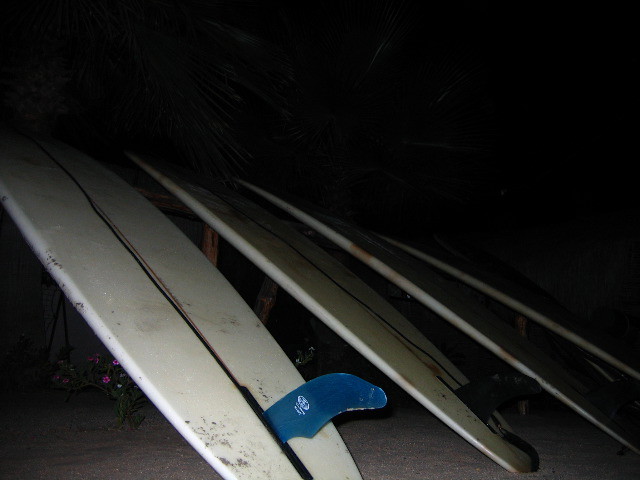The photograph, taken at night with flash, captures four surfboards propped diagonally against a wooden railing structure, with their fins pointing skyward. The surfboards have a striking appearance with white bodies accented by black and red lines running down their centers. The two surfboards on the left are particularly more visible due to their darker colors—one predominantly dark blue, and another entirely black. The fins are prominent and feature unique designs, though barely discernible due to the low light. The ground underneath appears to be a mix of dirt and gravel, and clusters of purple-pink flowers are peeking through. Overall, the image is shrouded in darkness, making the details difficult to discern, except for the elements illuminated by the camera's flash. In the obscured background, faint silhouettes of palm trees can be just barely made out.